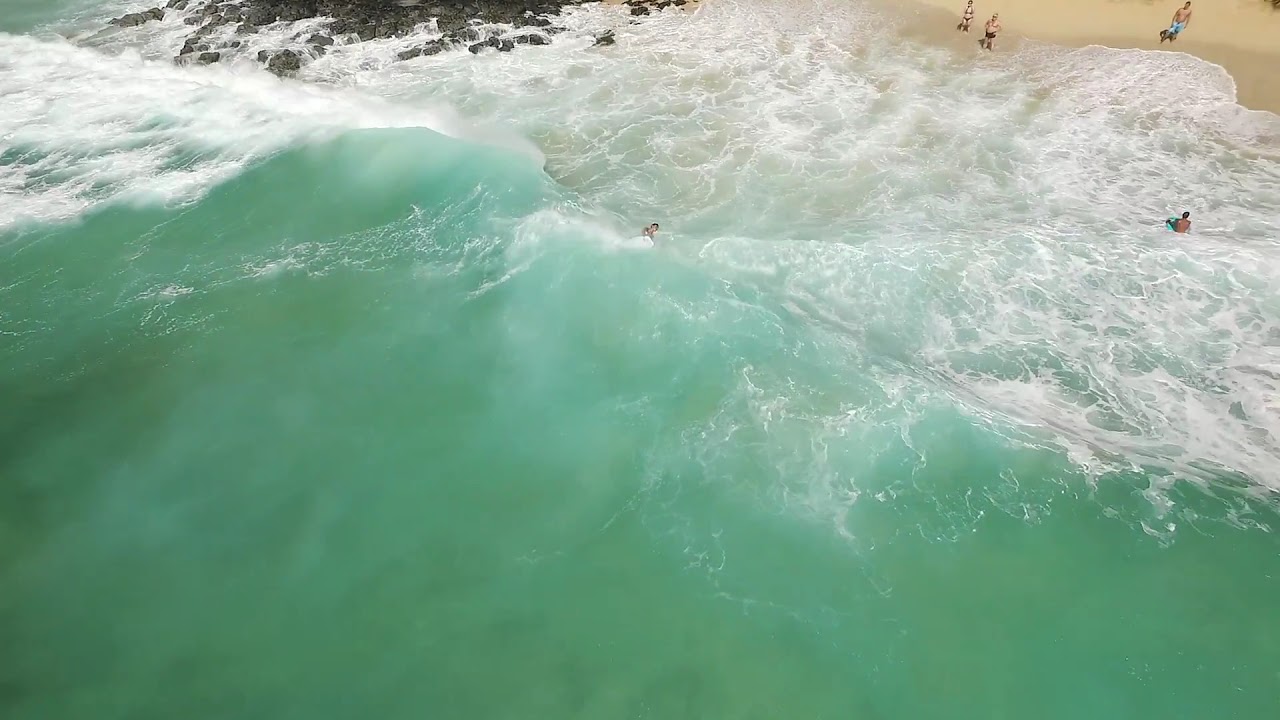This horizontally rectangular, full-color aerial photograph captures a lively beach scene bathed in bright, warm sunlight on a hot day. Taken from a low-flying vantage point, possibly a helicopter, the image predominantly features the green waters of the ocean, characterized by crashing waves and white foam indicative of a shoreline. In the upper right corner, a sliver of sandy beach is visible where three people are standing, while two others wade in the shallow water, hinting at attempts to surf or merely enjoy the sea. Black rocks occupy the upper left corner, adding texture to the scene. The varied colors of the image—white, gray, green, tan, red, and brown—enhance the vivid, sunlit atmosphere of a day spent outdoors by the ocean.